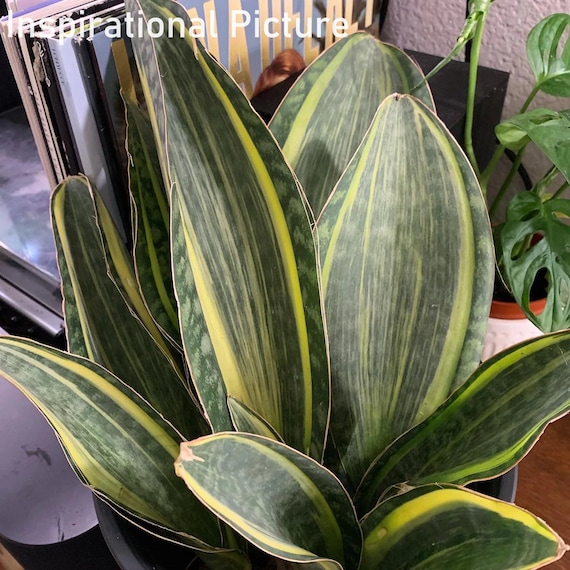This is a color photograph of a large, mostly green aloe vera plant with yellow and white variegated stripes, captured very close-up, likely inside someone's home. The plant is placed in a pot and positioned on what seems to be a wooden table or a bookshelf, with several books visible to its left. Behind the aloe vera, there is a smaller green plant in a white pot, possibly a philodendron, with multiple holes in its leaves, indicating it has not been well cared for. A portion of the wall, which appears to be white, is also visible in the background. The photo features two words at the top left that read "inspirational picture," although the image itself is simply a detailed close-up of houseplants in a domestic setting.